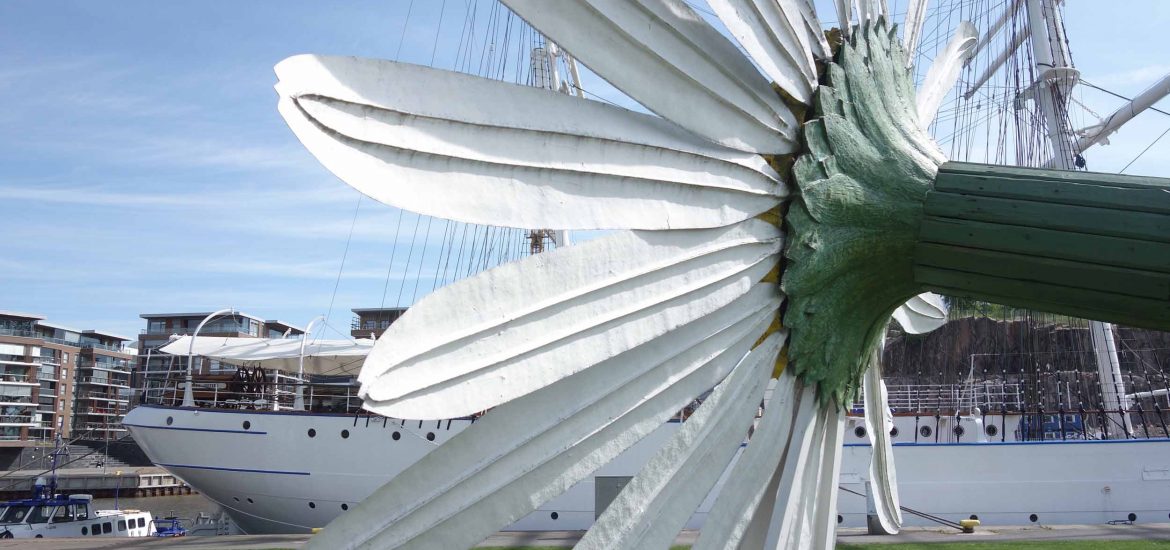The photo, seemingly an amateur shot taken from a boat or near a dock, features a large white ship with blue accents in the background, partially obscured by a massive sculpture that resembles a daisy. The sculpture boasts a green stem-like structure and several artificial white petals with a yellow centerpiece, mimicking a flower. Behind this intriguing sculpture, the ship appears significant in size, likely not a privately-owned vessel. The scene is set against a backdrop of various multi-story buildings in shades of brown, white, and black, under a blue sky dotted with fluffy clouds. Smaller boats are also visible, emphasizing the harbor setting. The daisy-like sculpture prominently dominates the foreground, making it challenging to see the entirety of the ship and adding a unique element to the urban landscape.